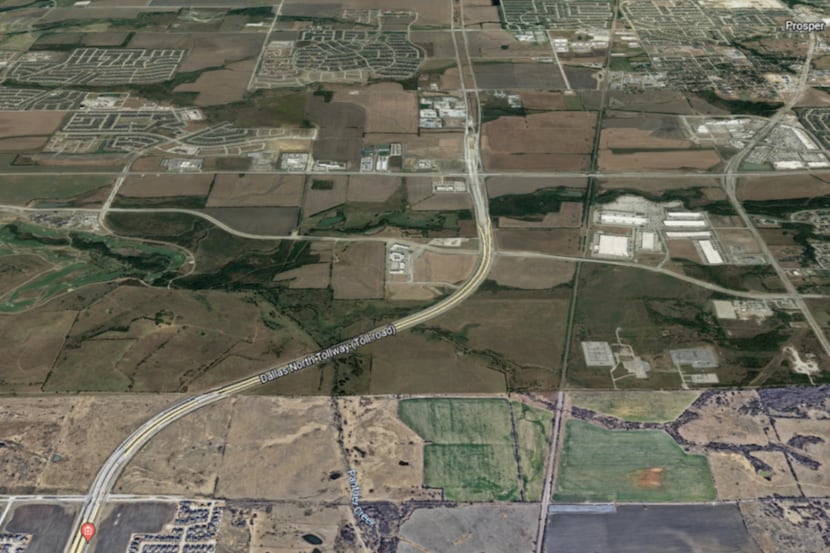The image is a full-color, square aerial photograph taken in the daytime, likely from an airplane, capturing a rural area with a blend of green fields, tan and brown barren lands, and scattered small buildings. Key digital enhancements include a red dot with unreadable white text in the lower left corner, which sits over the Dallas North Tollway (Toll Road). The upper right corner is marked with the word "Prosper." The image shows a distinct, grid-like pattern of roads and land parcels, likely indicating farmland. The scene, devoid of metropolitan density, suggests a location in Texas, inferred from the labeling of the Dallas North Tollway.